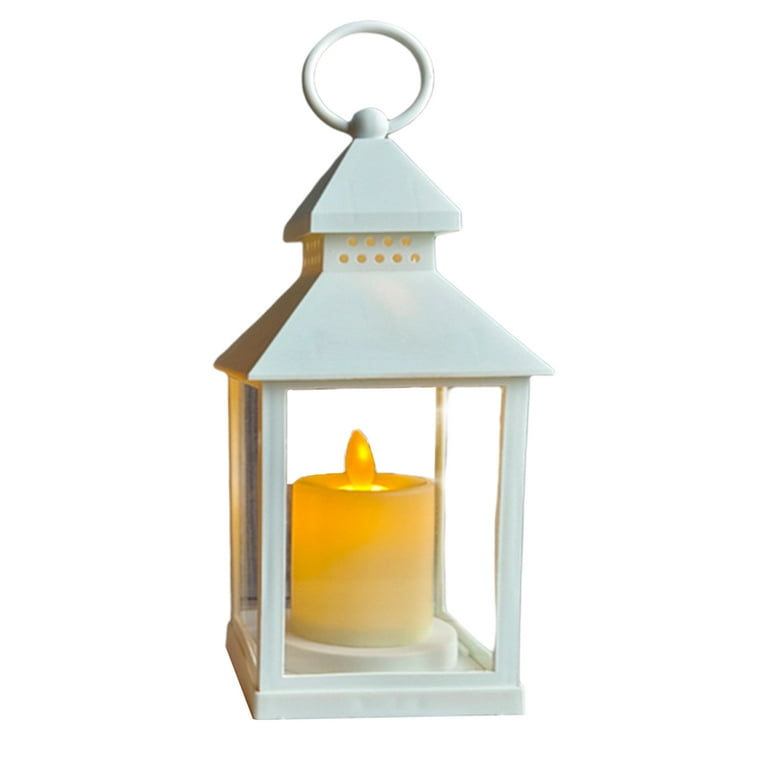The image features a white lantern styled like a birdhouse with a square base and transparent glass walls on all sides, allowing a clear view of the contents. Inside the lantern is a small, artificial candle with bright orange, yellow-colored wax, and an orange flame tipped with a white dot, likely an LED light, creating a cozy glow that illuminates the interior. The lantern has a distinctive architectural design with two sloped, arched roofs stacked atop each other. The uppermost part of the roof features a series of tiny holes arranged in neat rows, allowing light to escape and enhance the glowing effect. At the very top, the lantern is completed with a decorative round ball and a circular ring, making it easy to hang. The background of the image is completely white, emphasizing the lantern's intricate details and luminous ambiance.